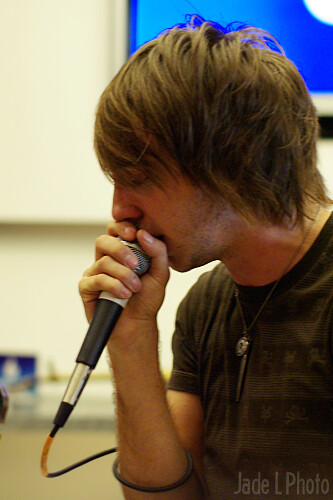In this detailed close-up image, a man is intensely singing into a microphone. Captured from his side profile, he is facing the left, with his right hand clutching the mic closely, such that it covers part of his mouth. His eyes are downcast in concentration, exuding a sense of deep emotion. He has shaggy, dark brown hair styled in side-swept bangs reminiscent of early 2000s fashion, partially concealing his ear. His facial hair is slightly stubbly, and he sports a distinctive black shirt with subtle gray stripes, complemented by a silver necklace with a pendant. The microphone cord is wrapped around his arm, adding to the dynamic intensity of the moment. The background is blurred, hinting at an indoor setting, possibly a recording studio or a church with a modern rock vibe, marked by a nondescript wall and a monitor likely displaying a blue screen. At the bottom of the image, a watermark reading "Jade L Photo" is visible, attributing the photographer.